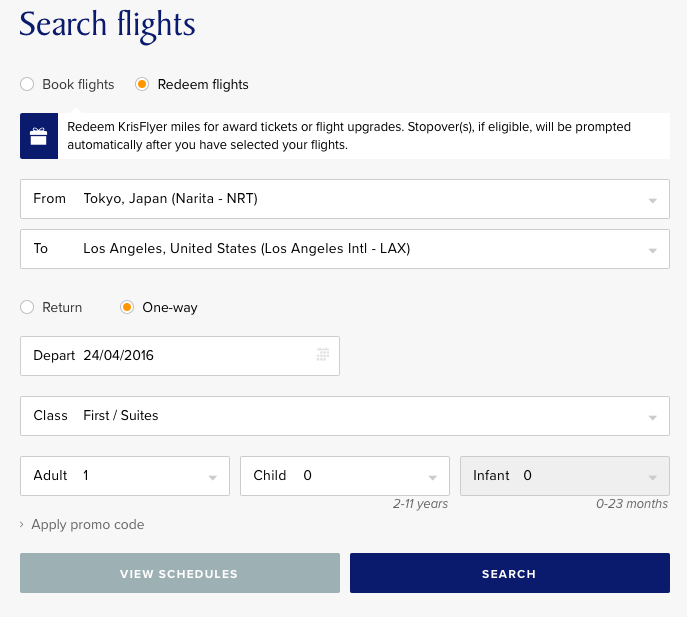**Caption:**

A screenshot from an airline website displays a booking form with a gray background. In the upper left corner, a blue banner reads "Search Flights." Below are two toggle options: "Book Flights" and "Redeem Flights," with the latter selected and highlighted by an orange circle. A blue box with a white gift icon appears, explaining, "Redeem KrisFlyer miles for award tickets or flight upgrades. Stopovers, if eligible, will be prompted automatically after you've selected your flight."

The form starts with two fields: "From" and "To." The "From" field shows "Tokyo, Japan, Narita (NRT)" with a dropdown arrow, and the "To" field shows "Los Angeles, United States, Los Angeles International (LAX)" also with a dropdown arrow. The next option offers a choice between "Return" or "One Way," with "One Way" selected.

The "Depart" field indicates the date "24/04/2016." The class selection shows "First/Suites" with a dropdown menu available. Passenger details are filled in as "1 Adult," with "0 Child" and "0 Infants," with the "0 Infants" option grayed out. At the bottom of the form, there's a section to "Apply Promo Code."

Two buttons conclude the form: a gray "View Schedules" button on the left and a "Search" button with white font on the right.